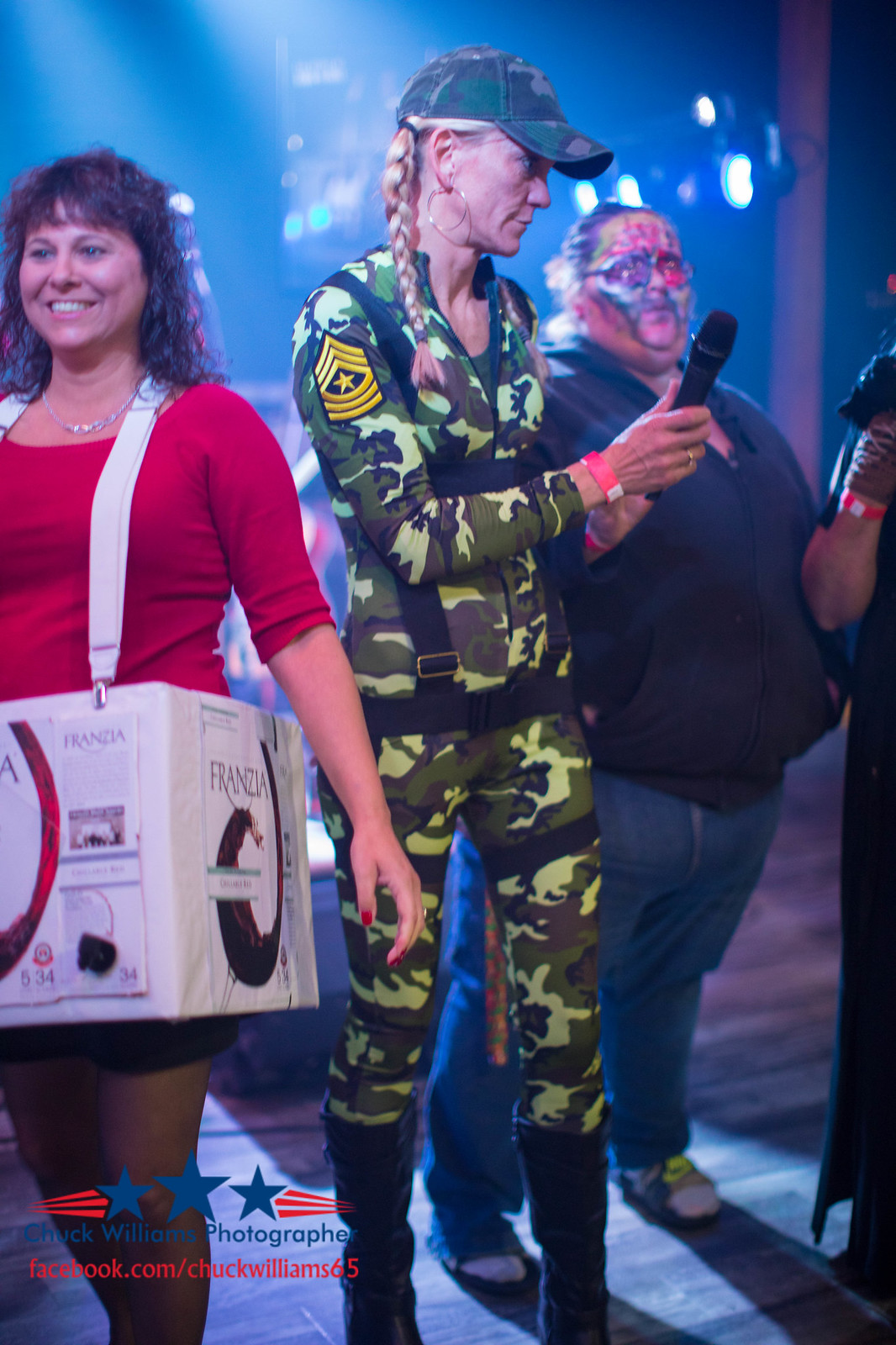In this photograph, set in a dimly lit building adorned with specks of light on the wall in the background, three women are pictured celebrating what appears to be Halloween. The woman in the center is dressed in a green camouflage outfit, complete with a camo hat and black boots. Her blonde hair is styled in braids, and she is accessorized with large silver hoop earrings. She holds a black microphone, turned sideways, in her hands. A yellow star badge is visible on her right shoulder.

To her left, partially cut off from the frame, is a woman with shoulder-length curly brown hair and bangs. She is wearing a red, elbow-sleeve-length top and a chain necklace. A white strap loops around her neck, holding a white box with the branding "Franzia," indicating her costume as a box of wine. She is smiling and looking to the left, with blue eyes and a cheerful expression.

On the right side, slightly in the background, stands a heavyset woman with her hair pulled back, adorned with intricate blue and red face paint. She wears a dark top paired with blue jeans.

In the lower-left corner of the image, a darkened logo featuring three blue stars with red stripes can be seen, indicating the photograph credit: Facebook.com/ChuckWilliams65.